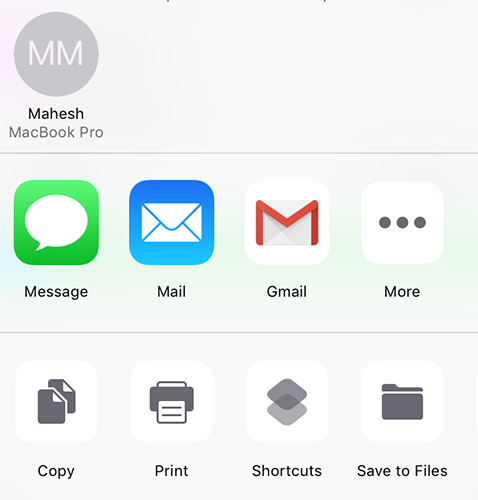This image is a screenshot captured on someone's cell phone. In the top left-hand corner, there is a gray circle with two capital M's next to each other, indicating the user "Mahesh," spelled M-A-H-E-S-H. Directly below this, "MacBook Pro" is displayed, with each part of the name capitalized as "M, A-C, B-O-O-K, P-R-O."

A faint gray line spans horizontally across the screen below the "MacBook Pro" text. Moving further down, various icons can be seen, each representing an app or action:

1. A green square containing a white speech bubble labeled "Message."
2. A blue square with an envelope labeled "Mail."
3. A white square with an envelope outlined in red labeled "Gmail."
4. A white square with three horizontal dots labeled "More."

At the bottom of the screen, several actions are displayed:

1. Two overlapping papers labeled "Copy."
2. A printer icon in a box labeled "Print."
3. Two diamonds in a box labeled "Shortcuts."
4. A file folder icon labeled "Save to Files."